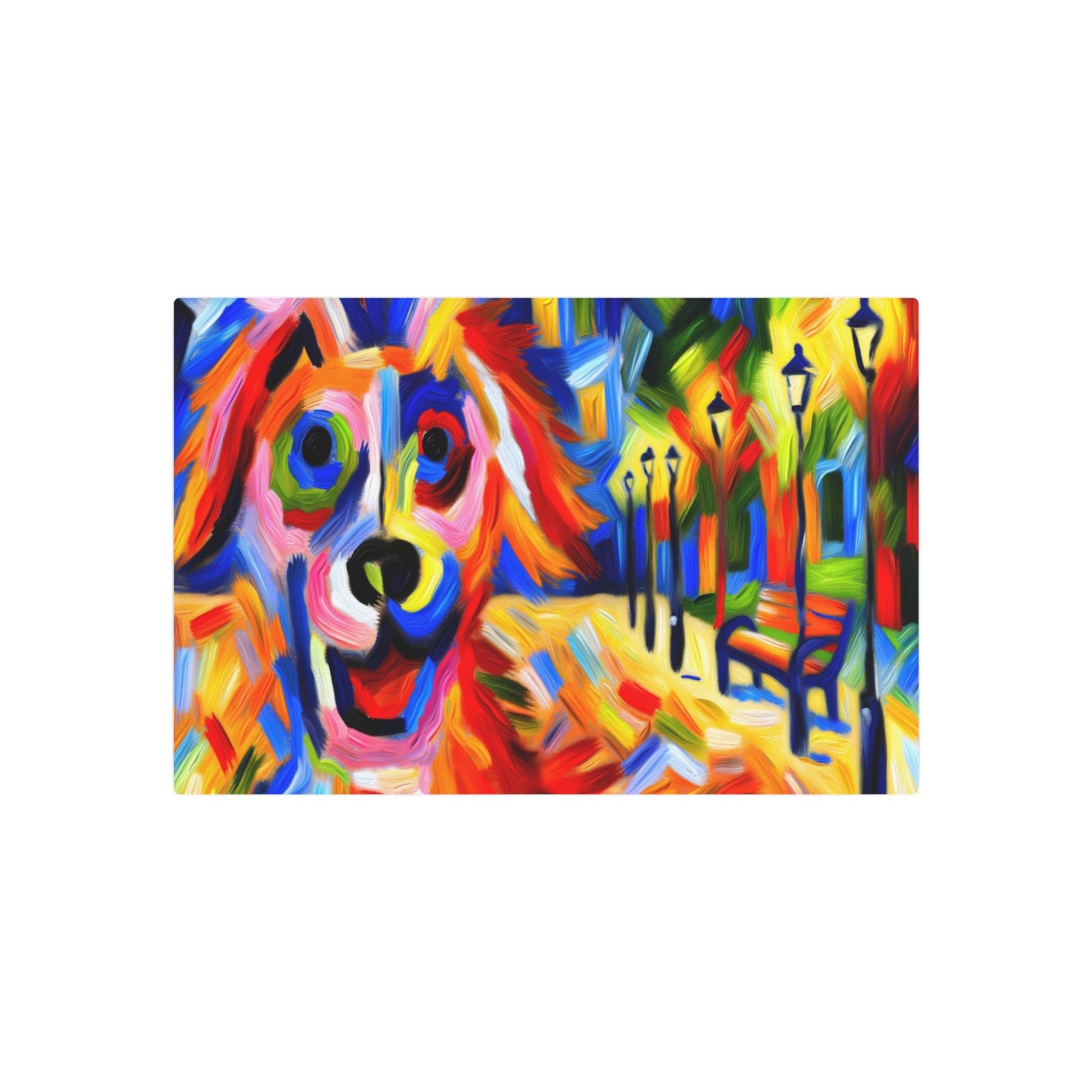The vivid painting is an abstract, rectangular artwork rich in vibrant hues. On the left side of the canvas, a partial depiction of a dog dominates the foreground. The dog’s head and upper torso are awash with a kaleidoscope of colors including green, blue, pink, yellow, red, and orange. Its nose is primarily black with splashes of yellow, while the areas around its eyes and ears blend shades of red, blue, green, yellow, black, orange, and pink. The dog’s tongue is a mix of pink and light blue, and its chest is dappled with colors ranging from orange to white to light blue to dark blue to red and green.

On the right side of the painting, the background features a series of six black street lamps topped with yellow lights, casting a soft glow. Below, a park bench with a black outline and brown wooden slats sits on a yellow walkway. Behind the bench, a blue building with a green lawn adds depth. Despite these identifiable features, the entire scene is bathed in a burst of bright, non-traditional colors, giving the painting a dreamlike and imaginative quality. The space between these elements and the general image seems vast, possibly set against an all-white background, enhancing the abstract and fragmented nature of the artwork.